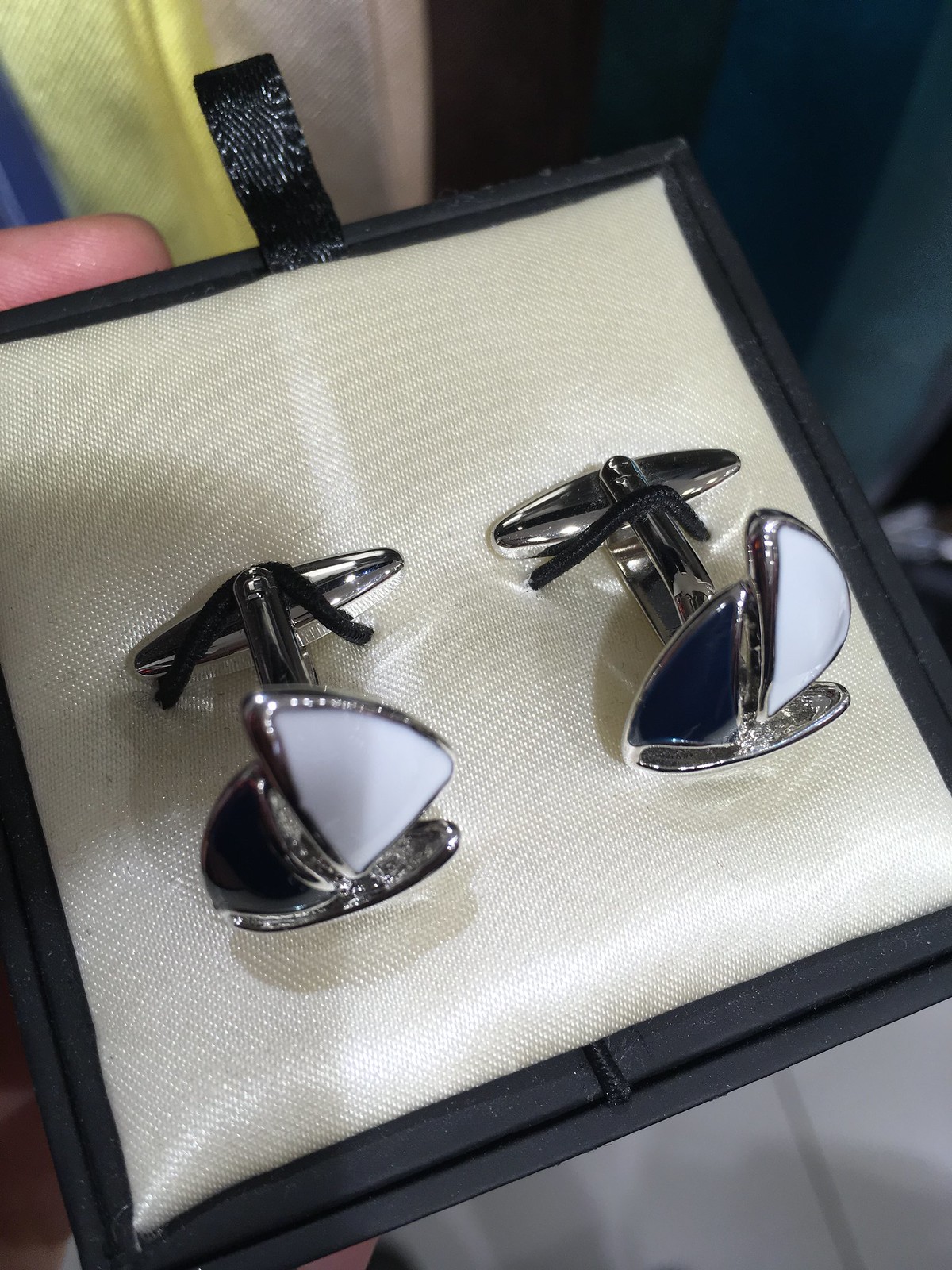The photograph features a black, square jewelry box, held by a person whose fingers peek into the frame. The box contains either a pair of earrings or cufflinks, each with a distinctive design. The jewelry inside is made of sterling silver with a sailboat or triangular motif—one element is white, while the other is navy blue. The inside of the box is cushioned with a beige or white fabric, appearing slightly pillowed. The background showcases a variety of colored fabrics, including stripes or panels of blue, yellow, white, and green, reminiscent of a gown. The lower portion of the image reveals a gray or white tile floor. The box is slightly angled with the right corner tilted upwards, enhancing the focus on the intricate details of the jewelry.